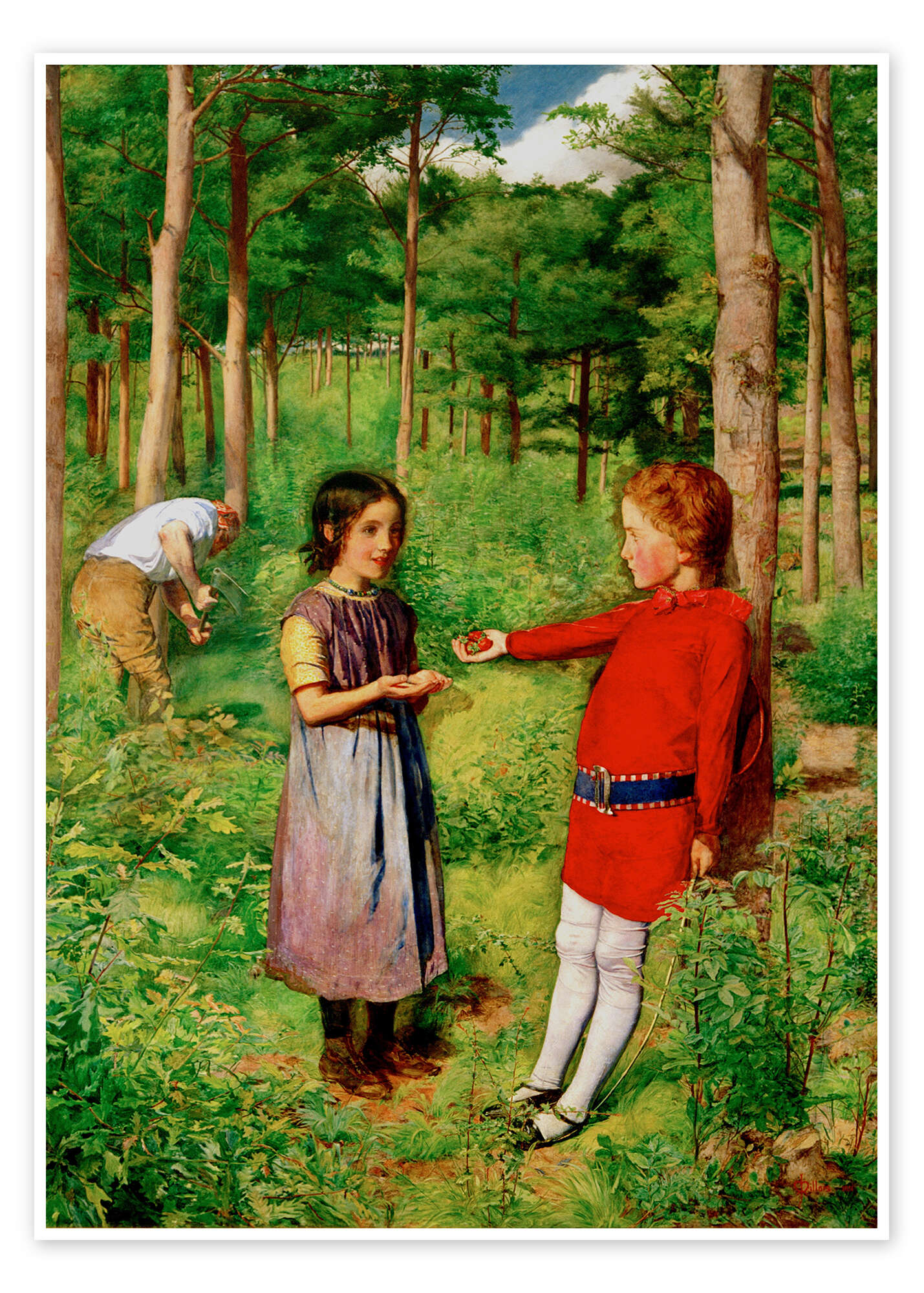This highly realistic painting captures a serene forest scene with three individuals in the foreground. At the center, a figure—potentially a man or woman—digs into the ground. Clad in a white t-shirt and khaki pants, the person’s face is not visible as their back is turned to the viewer. A hint of something reddish, possibly hair or a scarf, adds detail to their appearance. The object in their hand is ambiguous, possibly a shovel or another tool.

In the mid-ground, two children engage in a heartwarming interaction. A girl with short brown hair wears a charming purple dress over a yellow shirt, accented by a green necklace. Her hands stretch out towards a boy who, also red-haired, is dressed in a bright red outfit complemented by white leggings and black shoes. Leaning casually against a tree trunk, the boy offers strawberries from his right hand, which the girl eagerly reaches for.

The backdrop features a calming forest landscape with a modest dirt path meandering through the clearing, adding depth to this peaceful and inviting scene. The painting evokes curiosity about the purpose of the figure's digging, creating an overall atmosphere rich in narrative potential.